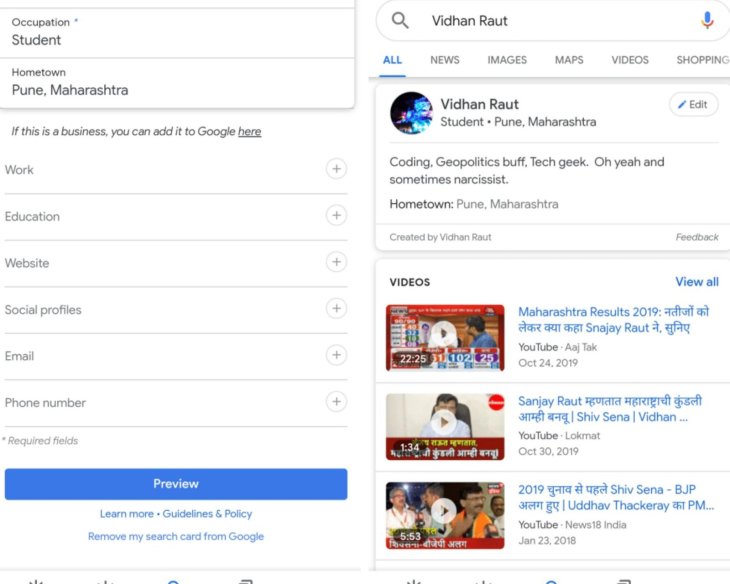In this image, the screen is split into two main sections. On the left side, the Google profile editor is displayed, showcasing various fields that can be filled out or edited. These fields include Occupation, Hometown, Work, Education, Website, Social Profiles, Email, and Phone Number. There is specific text filled in for the student field, indicating "Maharashtra, Hildon Pune, Maharashtra."

On the right side of the screen, the Google search results for the query "Vidhan Raut" are shown. The snippet of Vidhan Raut's profile mentions that he is a "Coding and Geopolitics buff, tech geek, oh yeah, and sometimes narcissist." Additionally, the search results include links to several YouTube videos, which are related to Maharashtra politics. The combination of these elements provides a comprehensive view of both the editable profile information and the public search results for Vidhan Raut.